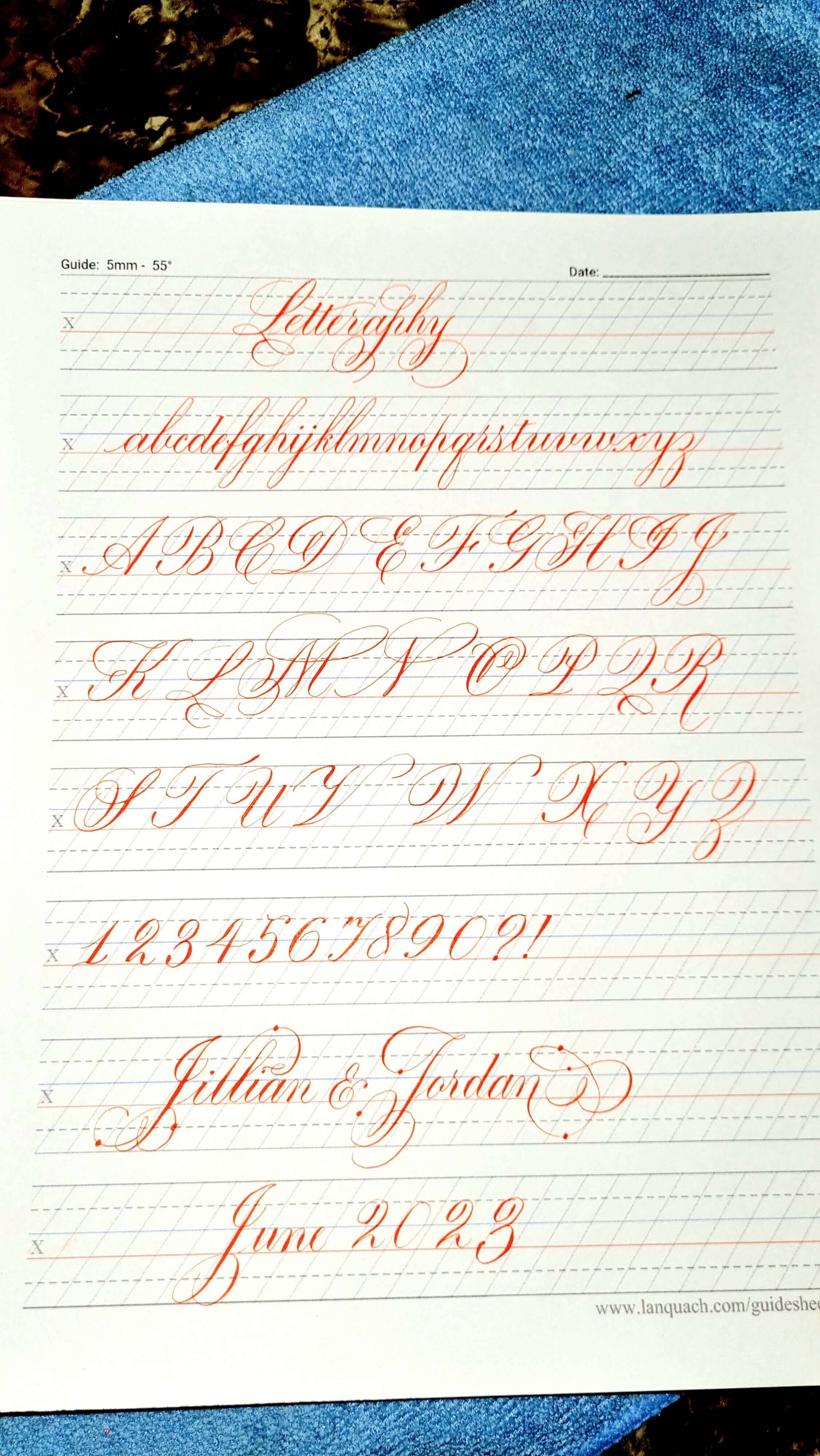The image features a sheet of lined paper laid on a blue towel or table. At the top of the paper, it says "guide 5mm-55 degrees," with a space labeled "date" but no date filled in. The word "letterography" is written prominently. The sheet displays the entire alphabet in lowercase cursive script, with each letter connected elegantly on one line. Below it, the alphabet is shown again in uppercase cursive, each letter clearly spaced, showcasing their ornate twists and flares. Further down, the sheet demonstrates how to write the numbers 1 through 9, followed by zero, a question mark, and an exclamation point. At the bottom, written in cursive, are the names "Jillian and Jordan," along with the date "June 2023." The detailed presentation seems to serve as a guide for learning or perfecting cursive writing.